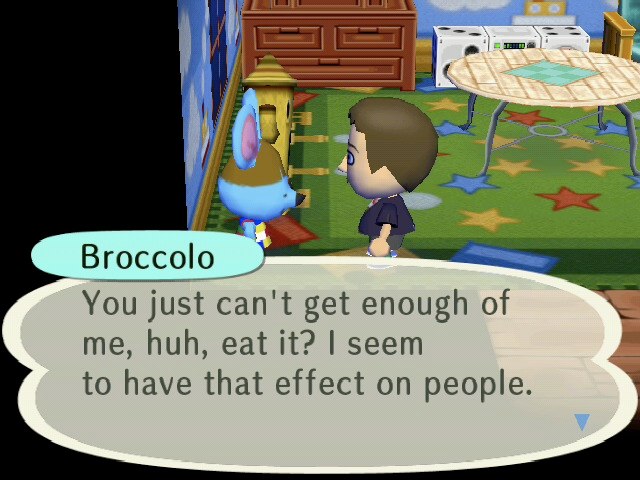This is a screenshot from a handheld video game, likely from the Nintendo Wii or similar console, and it resembles the style of Animal Crossing. The image captures a scene set in a kitchen-type room with a background predominantly black, contrasted by a vibrant, animated section on the right-hand side. The scene features a human character with dark gray hair, wearing a purple t-shirt, gray pants, and blue shoes, engaged in conversation with an animated blue mouse named Broccolo.

Broccolo, distinguished by his name in a smaller, blue-tinted dialogue box, is speaking to the human character. His dialogue is displayed in a larger, grayish, transparent speech bubble with a white border, stating, "You just can't get enough of me, huh? Eat it. I seem to have that effect on people." 

The room's floor is covered by a green carpet decorated with multicolored stars in blue, red, and yellow, as well as light blue dots. Central to the room is a round table with a wooden plank pattern and a green diamond-shaped design, supported by four curved legs. Behind the table stands a white music system, and a blue wall can be seen in the background. Additionally, a brown cabinet is positioned at the top-left, while an unidentified yellow object rests on the carpet's left-hand side.